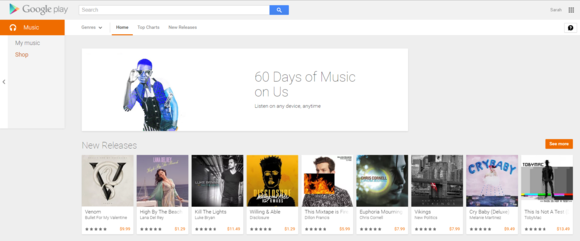The webpage displays the Google Play Store interface. At the top left of the page, the "Google Play" logo is prominently featured, accompanied by a white search bar directly beneath it. On the left side of the page, a navigation menu lists various categories, with "Music" highlighted in orange and marked with a headphone icon. 

Below the navigation menu is a horizontal white bar containing different menu options. The background of the page is a soft gray, providing a contrast to the content displayed. 

In the center of the page, there is a prominent white rectangle featuring an image of a man with vibrant blue hair, wearing a blue vest over a black button-down shirt. To the right of this image, a promotional message reads, "60 days of music on us."

At the bottom section of the page, there is a showcase of new music releases. This section displays nine album or song covers arranged in a grid format, each accompanied by a description. The vibrant album artwork and titles stand out against the gray background, inviting users to explore and download new music.